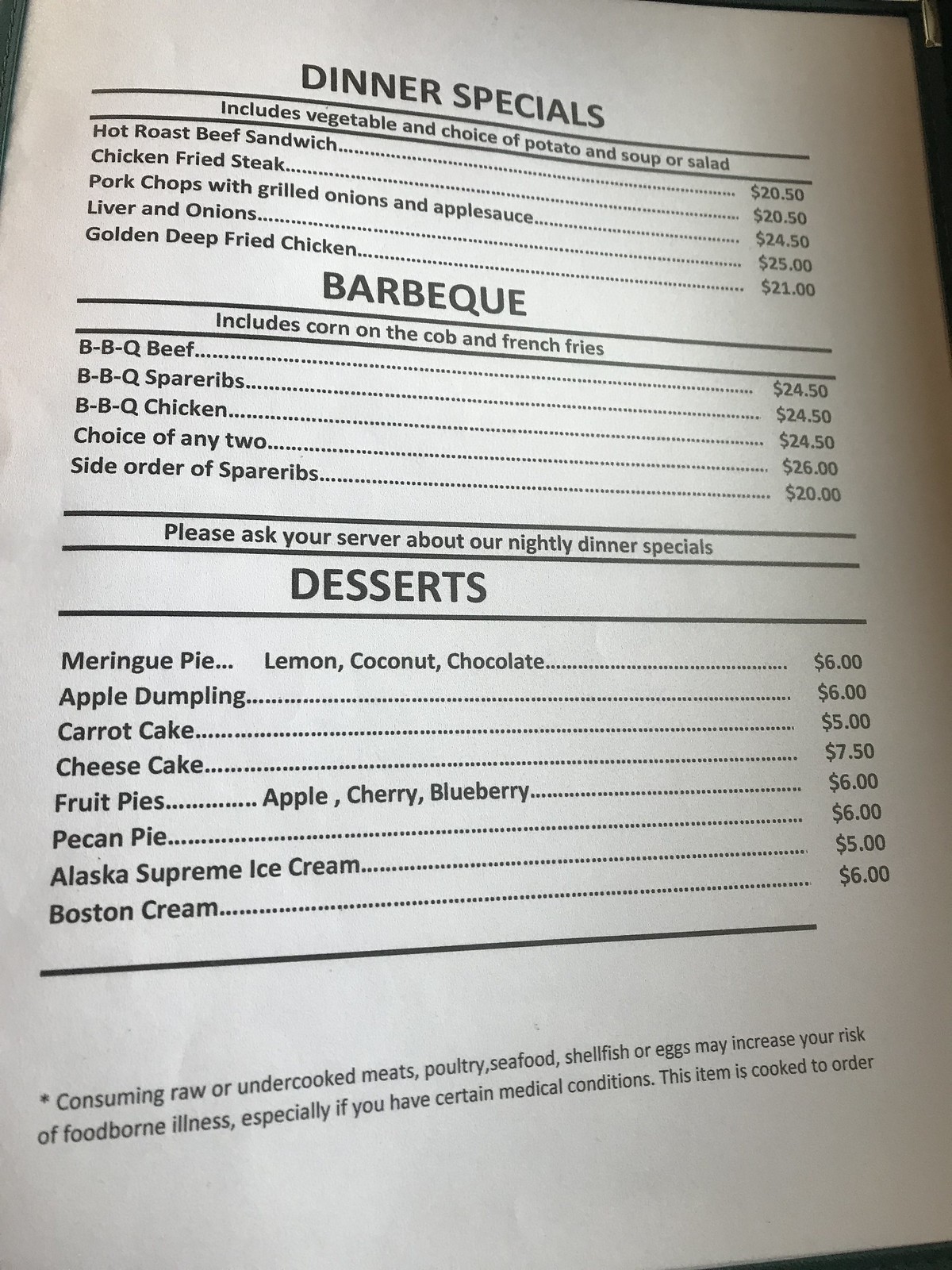The image captures a straightforward menu displayed on what seems to be a single sheet of paper. The layout is simple with plain black fonts on a white background, categorizing the offerings into three sections: Dinner Specials, Barbecue, and Desserts.

In the Dinner Specials section, patrons are informed that the meals come with vegetables, a choice of potato, and either a soup or a salad. The special dishes listed include:
- Hot Roast Beef Sandwich
- Chicken Fried Steak
- Pork Chops with Grilled Onions and Applesauce
- Liver and Onions
- Golden Deep-Fried Chicken

Moving to the Barbecue section, each entree is served with corn on the cob and French fries. The BBQ options and their prices are:
- Barbecue Beef: $24.50
- Barbecue Spare Ribs: $24.50
- Barbecue Chicken: $24.50
- Choice of Any Two Barbecue Items: $26.00
- Side Order of Spare Ribs: $20.00

Beneath the barbecue options, there is a note encouraging customers to ask their server about nightly dinner specials.

Finally, the Desserts section presents a variety of sweet treats, each priced as follows:
- Meringue Pie (available in lemon, coconut, or chocolate): $6.00
- Apple Dumpling: $6.00
- Carrot Cake: $5.00
- Cheesecake: $7.50
- Fruit Pies (apple, cherry, blueberry): $6.00
- Pecan Pie: $6.00
- Alaska Supreme Ice Cream: $5.00
- Boston Cream Pie: $6.00

Overall, the menu offers a clear and unadorned presentation of classic comfort food and indulgent desserts.